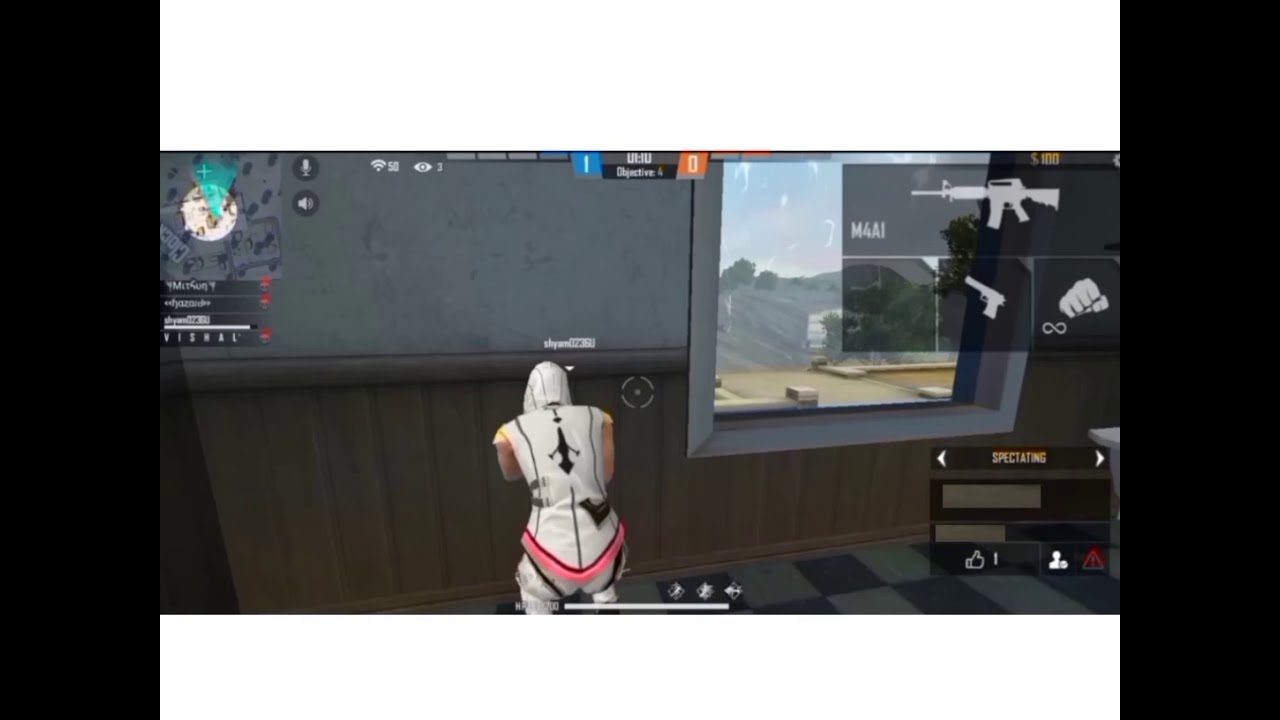The image is a highly detailed screenshot from a third-person video game, meticulously bordered by white strips surrounded by black strips on all four sides. The scene is set against a gray background with a brown wooden wall, reminiscent of wainscoting, and a checkerboard floor. The central focus is on a player character dressed in a skin-tight, white sleeveless jumpsuit with distinctive black markings and a pink belt. The character is seen from the back, crouched approximately three to four feet from the camera, which hovers about a foot above the character's head. 

To the right of the character, there's a large window through which various types of mountainous terrain are visible, adding depth to the scene. Above this window, a small panel displays two different guns and a closed fist, integrating essential GUI elements commonly seen in shooting arcade games. The sides of the image also feature additional GUI information, though the text is somewhat difficult to read. The image effectively captures the intricate blend of the in-game environment and the essential gameplay elements, highlighting the interactive and immersive nature of the game.